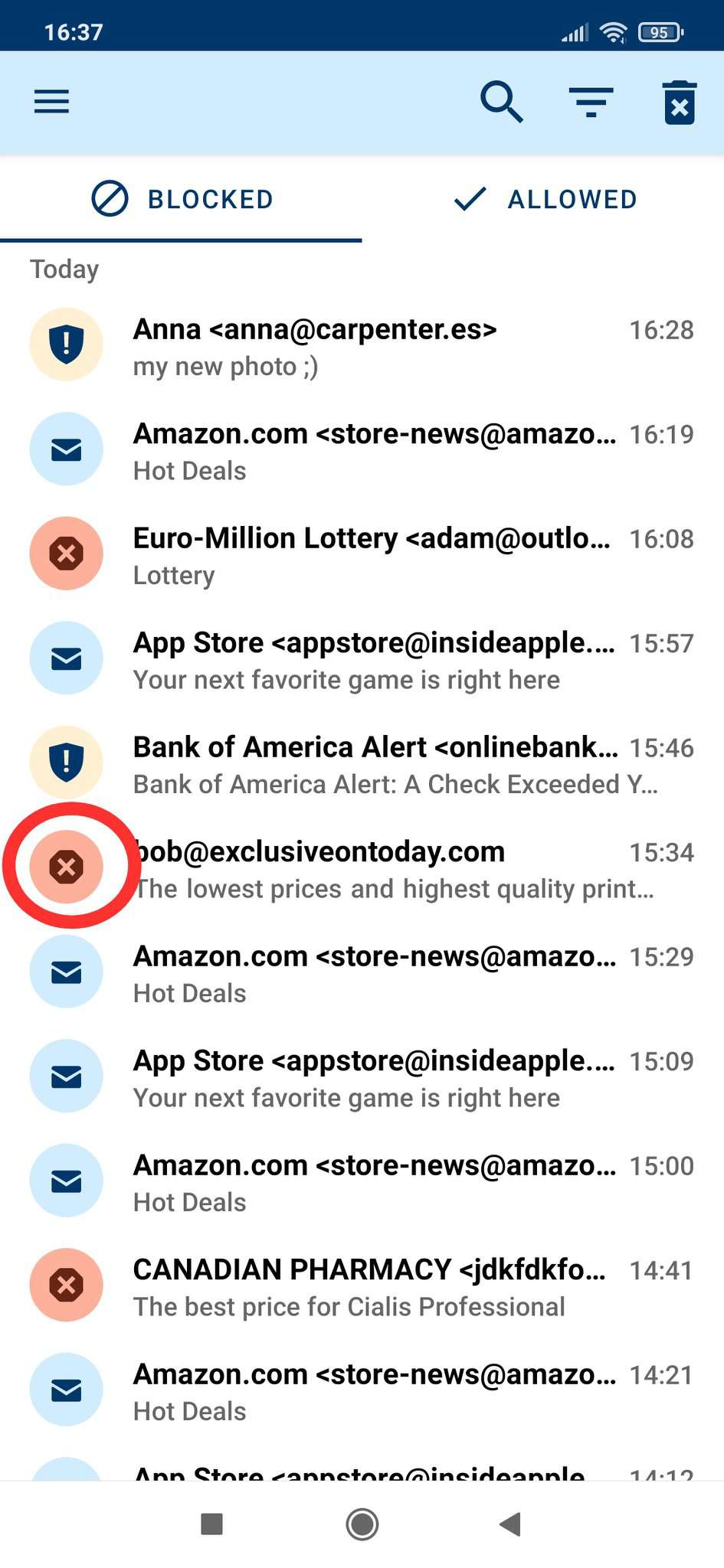The image is a screenshot from a smartphone displaying a list of allowed and blocked websites and emails. The top portion of the screen features a dark blue header panel showing the time, 16:37, with four to five signal bars, full Wi-Fi strength, and a 95% battery indicator. Below this, a lighter blue bar displays a hamburger menu icon on the left, a blue magnifying glass icon, a blue pyramid-like sorting icon, and a trash can icon.

Directly beneath this bar is a section divided into two columns: "Blocked" (indicated by a circle with a slash through it) and "Allowed" (indicated by a checkmark). Both sections categorize activities by date, starting with "Today."

The "Blocked" list includes around 11 or 12 entries, from the most recent downwards. The first blocked item, highlighted with an exclamation point badge, is an email from "Anna at Anna Carpenter dot ES" received at 16:28 with the subject "my new photo." Other blocked items include emails from "Amazon.com," "Stornews" (likely a newsletter or spam), and a phishing email with an octagon and cross icon titled "You're a million dollar adamant out something lottery." Further entries include alerts from the App Store and Bank of America. Notably, one email from "Bob at exclusive online today dot com" is emphasized with a red circle. Additionally, another item from a "Canadian pharmacy" is blocked.

The navigation menu is visible at the bottom of the screen, completing the interface.